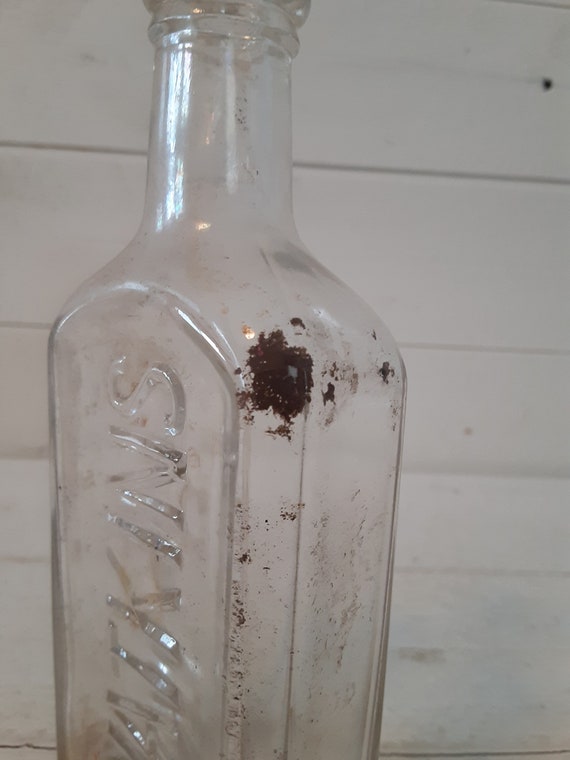A close-up image features a dirty glass bottle with significant caked-up dirt and scattered specks, particularly on the top portion near its narrow, rounded mouth opening and short cylindrical neck. The bottle, which has a square shape with rounded edges, appears to have text imprinted vertically down its side that reads "Watkins." Inside the bottle are indiscernible objects that may be bugs, given the odd shape of some contents. The background reveals a white wooden wall, marked with scuff spots, light patches, and a visible nail in the top right corner. The bottle is either standing on or in front of a surface, with the perspective possibly above the bottle, giving a clear view of both the wall and the dirt-streaked glass.